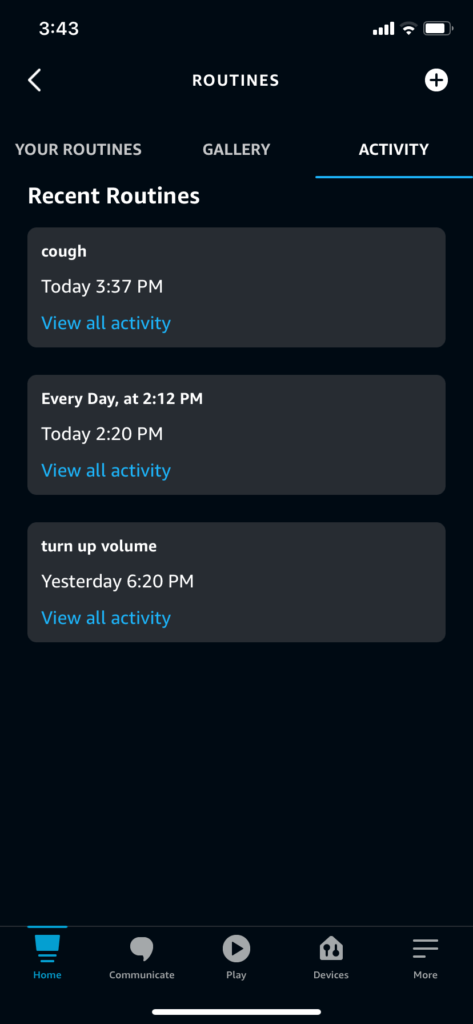The image is a screenshot of a smartphone's routines interface. At the top left, the time displayed is 3:04 PM. The top right indicates full cellular signal with four bars, the Wi-Fi signal at 2 out of 3 bars, and a battery level approximating 85%, though no percentage is explicitly shown. Just beneath this top bar, there's a left-facing arrow (greater-than sign) on the left, "ROUTINES" in bold white text at the center, and a black plus sign inside a white circle on the right.

The interface is divided into three tabs: "Your Routines," "Gallery," and "Activity," with "Activity" currently selected. Heading the active tab, we see "Recent Routines" in bold white font, listing three routines: "Today at 3:37 PM - Cough," "Everyday at 2:12 PM," and "Today at 2:20 PM - Turn up volume." At the bottom of the screen, there is a navigation bar with the icons and text for "Home," "Communicate," "Play," "Devices," and a "More" button.